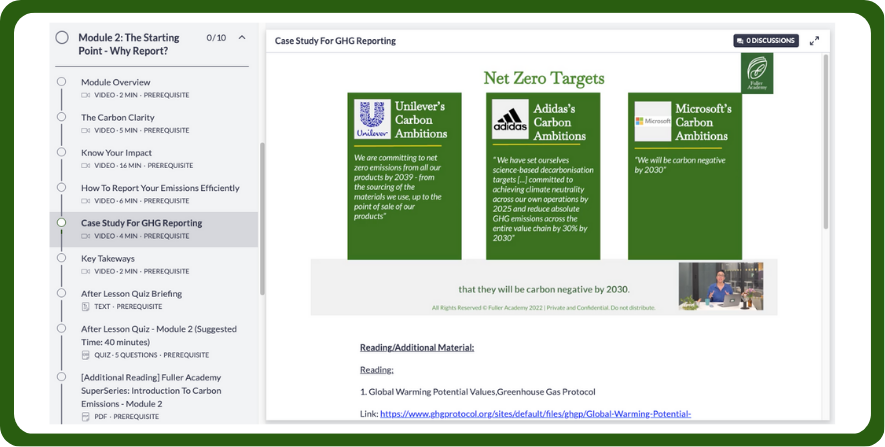**Caption:**

The image features a structured page layout with a distinct blue border on the left side and a white background. The left section of the page is titled "Module Two: Starting Point - Why Report?" and displays a progress list of included videos. The listed videos are as follows:

1. Module Overview
2. The Carbon Clarity: Know Your Impact
3. How to Report Your Imaging Efficiency
4. Case Study for GHG Reporting
5. Key Takeaways
6. After Lesson Quiz Briefing
7. After Lesson Quiz
8. Module 2 Suggested Additional Reading 

Additionally, there is a mention of the "Full Academy Super Series: Introduction to Carbon Emission."

On the right side of the page, against the white background, there's a detailed section titled "Case Study for GHG Reporting," which highlights three articles with green headers addressing "Net Zero Targets":

1. **Unilever Carbon Emissions**:
   - Unilever is committing to achieving net zero emissions from all products by 2039, covering the entire lifecycle from sourcing materials to the point of sale.
   - The background of the section is green, featuring the Unilever logo, a blue "U."

2. **Adidas Carbon Ambitions**:
   - Adidas has outlined its science-based decarbonization goals, targeting climate neutrality across its operations by 2025, and aims to reduce absolute GHG emissions across its entire value chain by 30% by 2030.
   - This section includes the black Adidas logo.

3. **Microsoft Carbon Emissions**:
   - Microsoft has pledged to be carbon negative by 2030, with repeated emphasis on this goal within the section.
   - The bottom segment indicates their strong commitment to this target.

At the bottom of the page, additional reading material is suggested, highlighting:
- "Global Warming Potential Values – Greenhouse Gas Protocols"
- An associated link, written in blue: [GHGprotocol.org](http://GHGprotocol.org)